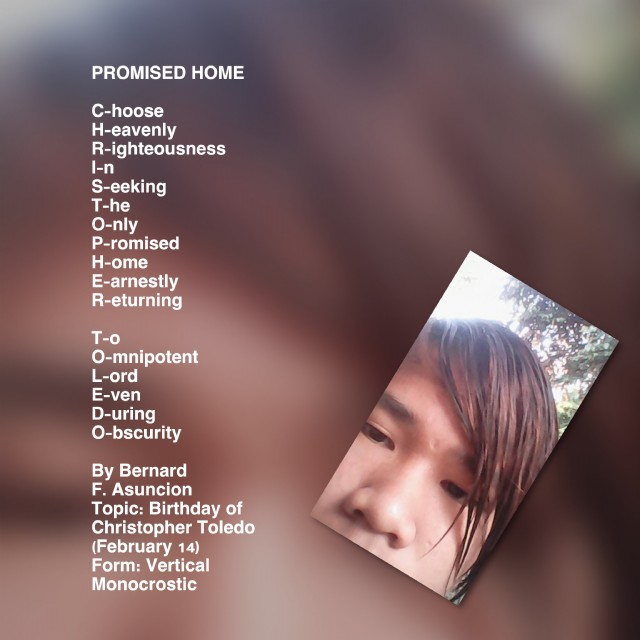The square image features a background with varying shades of brown, transitioning from a darker tone in the upper right to a lighter one in the lower left. Unpatterned and slightly blurred, the backdrop hosts a detailed, vertically aligned acrostic message on the left side in all caps white text. The text starts at the top left corner and extends to the bottom, reading "PROMISED HOME." Beneath this header, it spells out the name "Christopher Toledo," with each letter followed by a word: 

- C for Choose
- H for Heavenly
- R for Righteousness
- I for In
- S for Seeking
- T for The
- O for Only
- P for Promised
- H for Home
- E for Earnestly
- R for Returning

For Toledo:
- T for To
- O for Omnipotent
- L for Lord
- E for Even
- D for During
- O for Obscurity

The bottom of the text attributes the message to Bernard F. Asuncion with the topic mentioned as the birthday of Christopher Toledo on February 14th, formatted as a vertical monocrostic. On the right half of the image is an offset rectangular photo leaning towards the bottom right corner. The photo displays a close-up of an Asian teenager, presumably Christopher Toledo, with brown eyes, light skin, and straight brown hair swooping over the left side of his face. The top part of the photo features a blue sky with green trees, indicating an outdoor setting. The overall presentation suggests a heartfelt and inspirational religious message centered around Christopher's birthday.